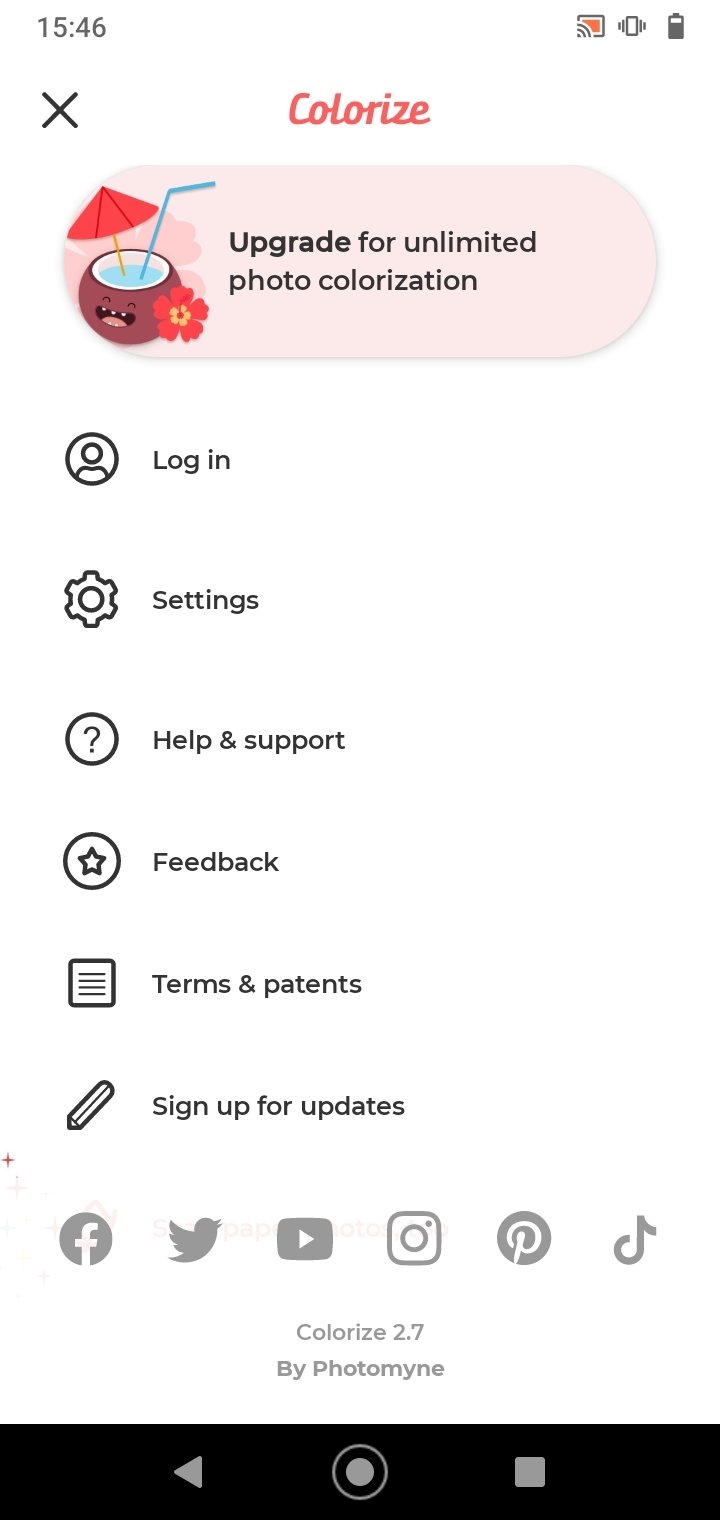This image, captured from the screen of a cell phone, exhibits a digital interface with the time prominently displayed as 15:46. On the right-hand side, three icons are visible, while the left side features an "X" mark. The word "Colorize" appears in a striking reddish hue.

Beneath this section, there is an illustration of a tropical coconut drink adorned with a small umbrella, straw, and a flower in the corner. Accompanying this image, a pink banner reads, "Upgrade for unlimited photo colorization."

The left side of the screen is lined with vertically arranged icons, each labeled with descriptive text. The bottom section of the display houses icons for various social media platforms, including Facebook, Twitter, YouTube, Instagram, Pinterest, and TikTok.

Near the very bottom, controls for navigation are present in a black rectangle, featuring a triangle pointing left, a clickable circle button, and a square. Just above these controls, options for "Login," "Settings," "Help and Support," "Feedback," "Terms and Patents," and "Sign Up for Updates" are neatly listed.